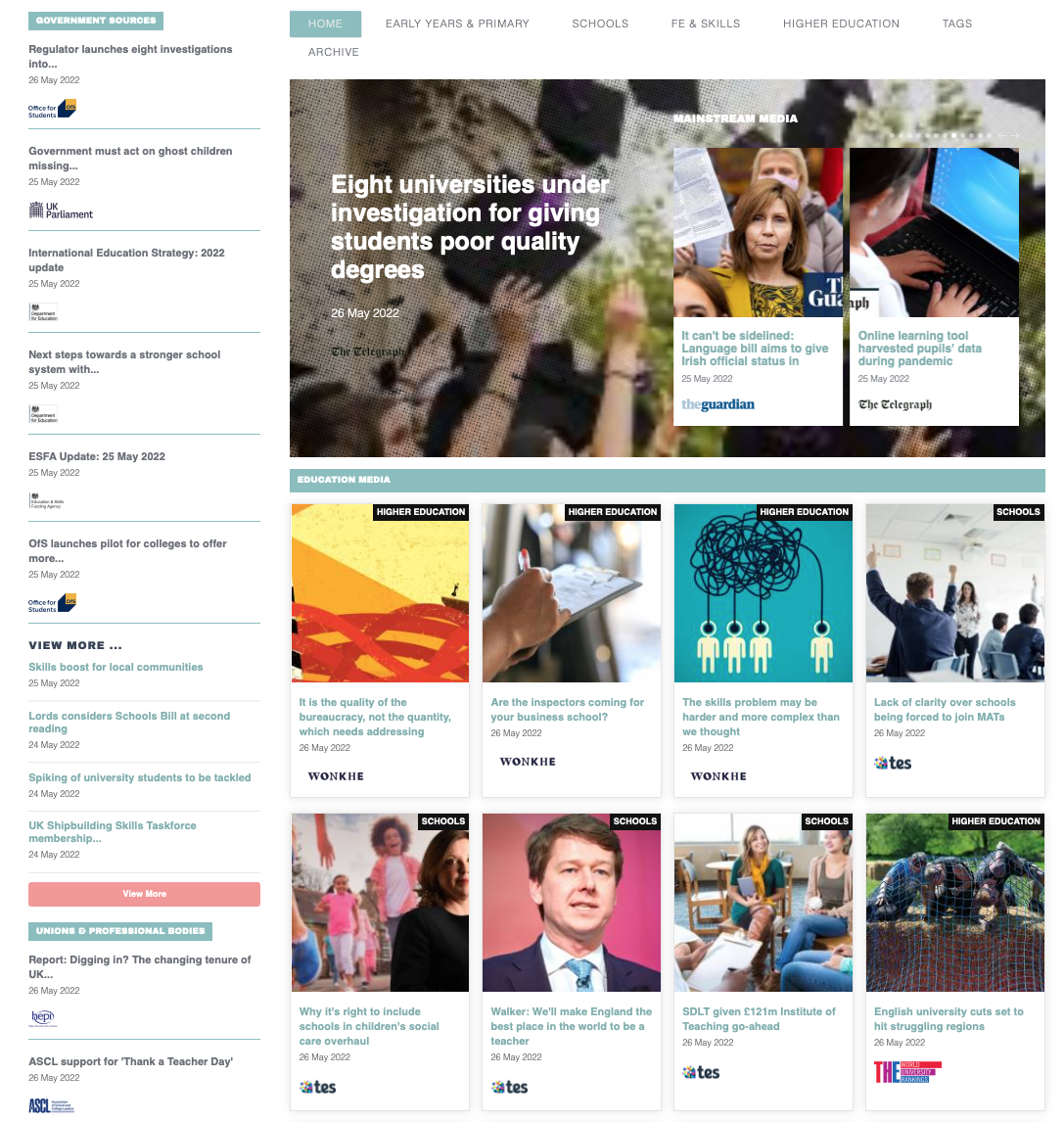**Detailed Caption:**

The screenshot showcases a news site with a focus on governmental and educational topics, though it’s somewhat ambiguous in its presentation. At the upper left corner, the text "government sources" hints at official content, while the site predominantly features news articles. 

The left-hand side of the page includes multiple headlines such as "Regulator launches aid investigations," "Government must act on ghost children missing," and "International Education Strategy 2022," suggesting a mix of regulatory and community-focused news. Further down, more topics related to community and educational issues are listed, reinforcing the site's apparent focus on news.

In the content section to the right, there's a main menu with categories like Home, Early Years, Primary Schools, FE and Skills, Higher Education, Tags, and Archive, indicating that the site likely specializes in educational content.

A prominent, albeit grainy and blurry, hero image depicts children celebrating by throwing their graduation caps into the air. Accompanying the image are two overlay panels: one headline, "Eight universities under investigation for giving students poor quality degrees," and another from The Guardian, "Language bill aims to give Irish official status."

Below, a smaller image shows someone using a laptop, with the caption “Online learning tools harvested pupils' data during pandemic,” sourced from The Telegraph. The page continues with eight more stories, each represented by a thumbnail image and a headline. The first three stories are marked "Higher Education" and the last one "Schools," again underscoring the focus on educational matters. 

Other thumbnails utilize stock photography and are associated with various publications such as The Guardian, Wonky, and TES, suggesting a diverse range of sources contributing to the content.